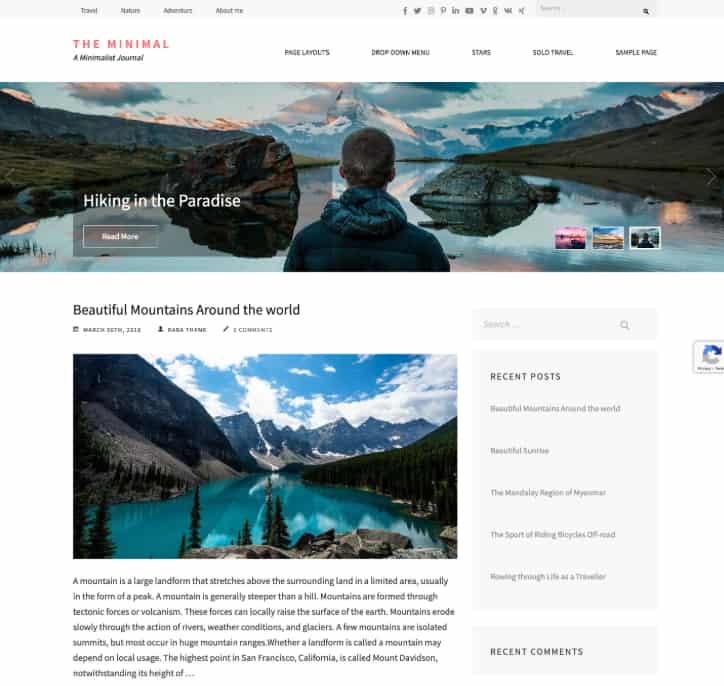In the image, the top section features a menu with four distinct options labeled "Travel," "Nature," "Adventure," and "About Me." The word "Minimal" is prominently capitalized in pink lettering. To the far right of the menu, there's a search icon and several clickable social media icons including Venmo, LinkedIn, YouTube, Pinterest, Twitter, and Facebook.

Directly beneath the "Minimal" heading, the site provides further navigation options with items labeled "Show," "Price," "Layouts," and a dropdown menu possibly labeled "Stars". There are additional categories such as "Solo Time" and "Sample Page."

The main image showcases a man standing with his back to the camera, wearing a hoodie. He overlooks a pristine body of water bordered by a few boulders. The scene is illuminated by a stunning sunset, setting behind distant mountain peaks, flanked by picturesque valleys. Below the image, the caption reads "The Beautiful Mountains Around The World."

Another similar image beneath it, devoid of any human presence, is dated March 2012 with a brief description accompanying it. To the right, there's a sidebar containing "Recent Posts" with about five options listed, followed by a "Recent Comments" section, which is currently empty. Above the "Recent Posts" section, a search bar is available for users to find specific content.